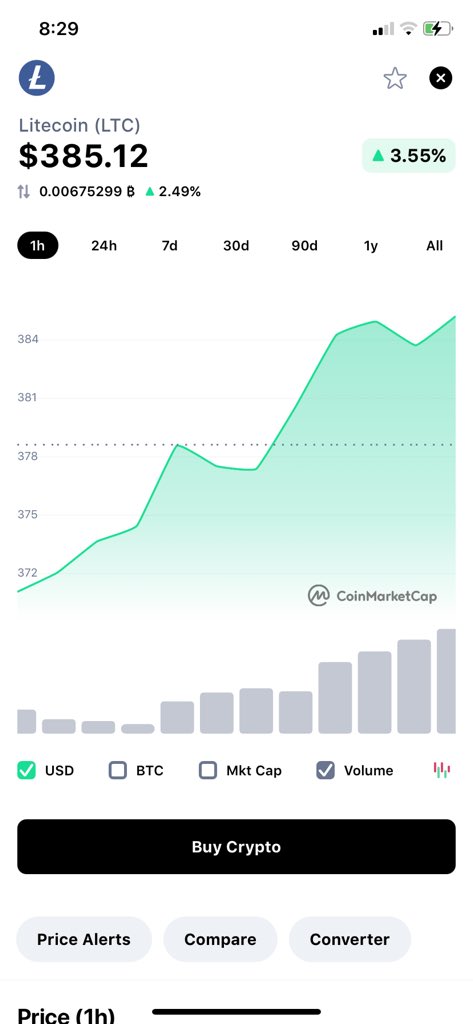The image displays a cell phone screen with several elements. In the upper left corner, the time is shown as 8:29. On the upper right, there are icons indicating cellular signal strength, Wi-Fi connectivity, and a green battery icon indicating that the device is charging. Below these icons, there is a white "L" in a blue circle, and to its right, a gray-outlined star followed by a white "X" inside a black circle.

Further down, the screen shows the current status of Litecoin (LTC): $385.12, up 3.55%. It also shows a volume metric of 0.00675299B, which is up by 2.49%, with this data being updated an hour ago. 

Below this information is a graph illustrating Litecoin's market cap, denoted in USD. The graph displays Litecoin's price movement starting from a low of $372 and rising to over $384. Next to the graph is a green box with a white checkmark labeled USD, and to its right, a gray box with a white checkmark labeled BTC.

At the bottom portion of the screen, there is a big black button with white text that says "Buy Crypto." Below this button, additional options read "Price Alerts," "Compare," and "Converter." The label "Price 1H" appears in parentheses, likely referring to price changes in the last hour.